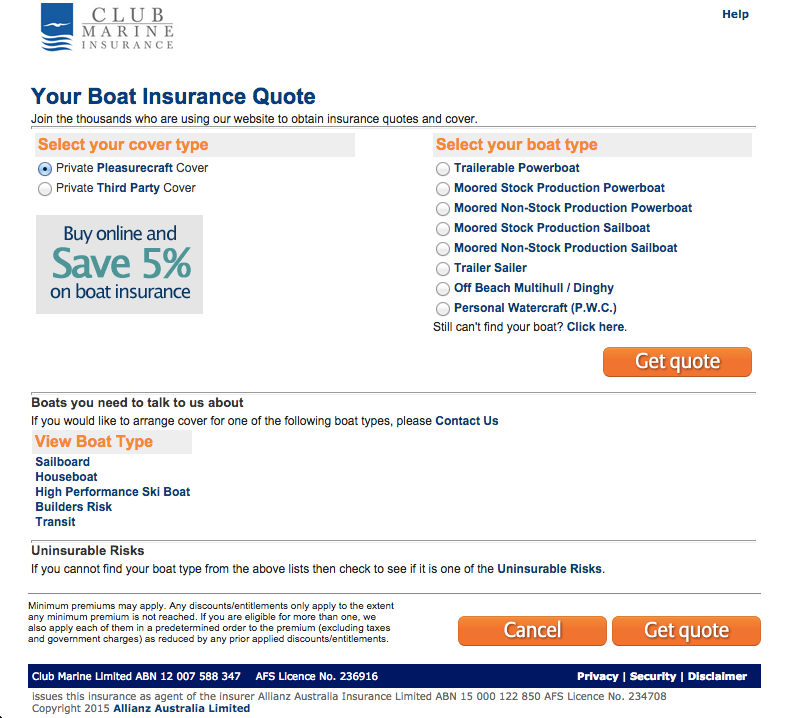Club Marine Insurance Poster: 

"Obtain Your Boat Insurance Quote Today!

Join the thousands who are already using our website to get their boat insurance quotes and cover. Select the type of coverage you need:
- Private Pleasure Craft Cover
- Private Third-Party Cover

Buy online and save 5% on your boat insurance!

Choose your boat type:
- Trawler
- Trailerable Power Boats
- Production Power Boats (stock or custom)
- Sailboats (stock or custom)
- Personal Water Craft (PWC)
- Dinghy

If you still can't find your boat type, click here.

Get a cool and comprehensive insurance quote now!"